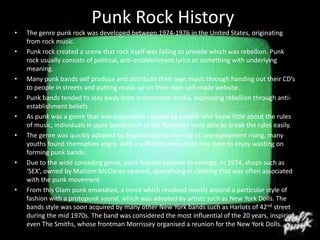The image features a nostalgic nod to retro technology, depicting an old curved television screen with a green glow, set against a black background. At the top, white text boldly announces "Punk Rock History," introducing a bullet list of information about punk rock. This list consists of eight bullet points in small white font, difficult to read due to the screen's glare. In the lower right corner, the iconic "Daft Punk" is mentioned, although partially obscured. The scene captures a fusion of vintage tech and punk rock information, framed within the glowing, low-quality screen reminiscent of thick, glass-fronted monitors from past decades.